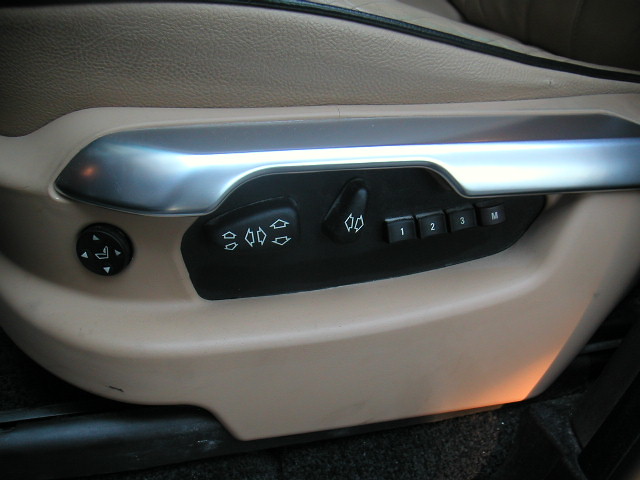The image depicts a close-up of the driver's seat interior of a car, focusing on the control panel on the side of the seat. The seat is upholstered in cream-colored leather, transitioning into a tan molded plastic towards the controls, with a metallic silver armrest feature. Prominently visible are the seat adjustment buttons, detailed with white directional arrows. These include a central circular button for multi-directional movement (up, down, left, right), as well as additional individual buttons for specific adjustments: one with arrows for vertical and horizontal tilting; another for seat back adjustments marked with left and right arrows. Further to the right are buttons labeled with numbers one, two, and three, alongside an 'M' button, likely used for preset seating positions. The plastic lining around the controls appears slightly dirty, and there is a pale light illuminating the bottom right corner, adding a subtle glow to the detailed setup.